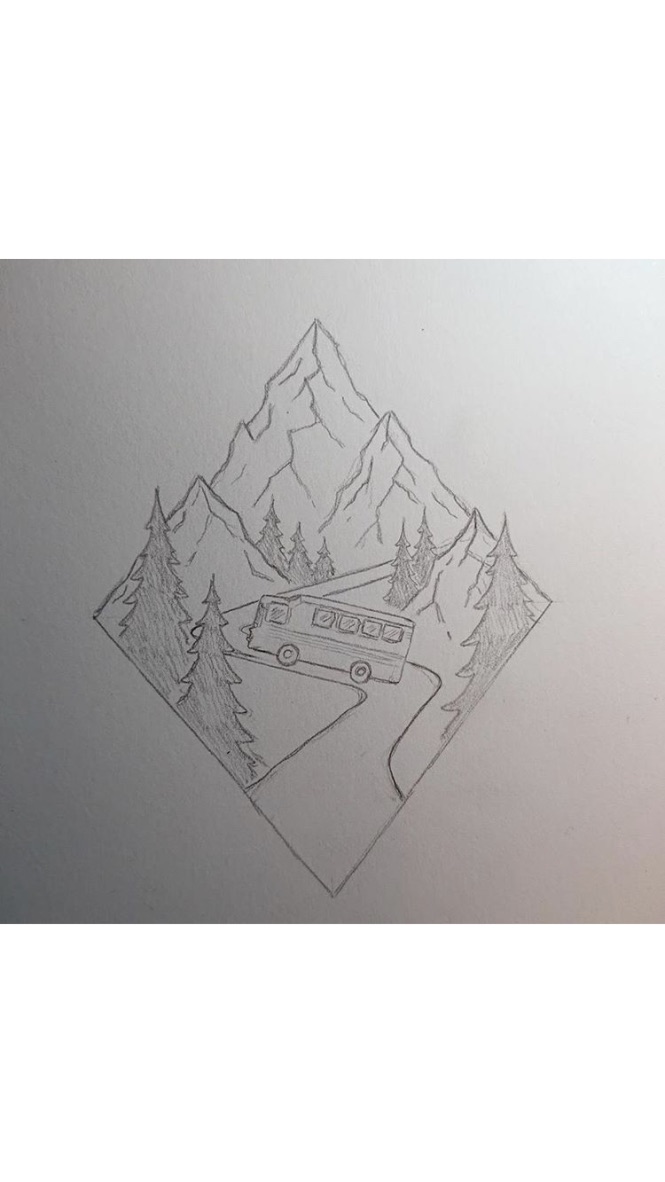A meticulously detailed line drawing on white paper, possibly hand-drawn, is depicted in a diamond-shaped format. The topmost point of the diamond showcases a prominent mountain, overlapped by two additional mountains reaching towards the right and left. At the heart of the drawing, where all three mountains converge, the outlines of three distinct evergreen trees are visible. Two trees are situated at the left point of the diamond while one stands at the right point. Near the winding road, leading from the bottom point of the diamond past the right mountain, two more evergreen trees are sketched. Traversing this road is a rectangular RV with four visible windows along its side, rounded edges, and two clearly defined wheels. The dark tones add a subtle ambiguity, enhancing the drawing's captivating intrigue.